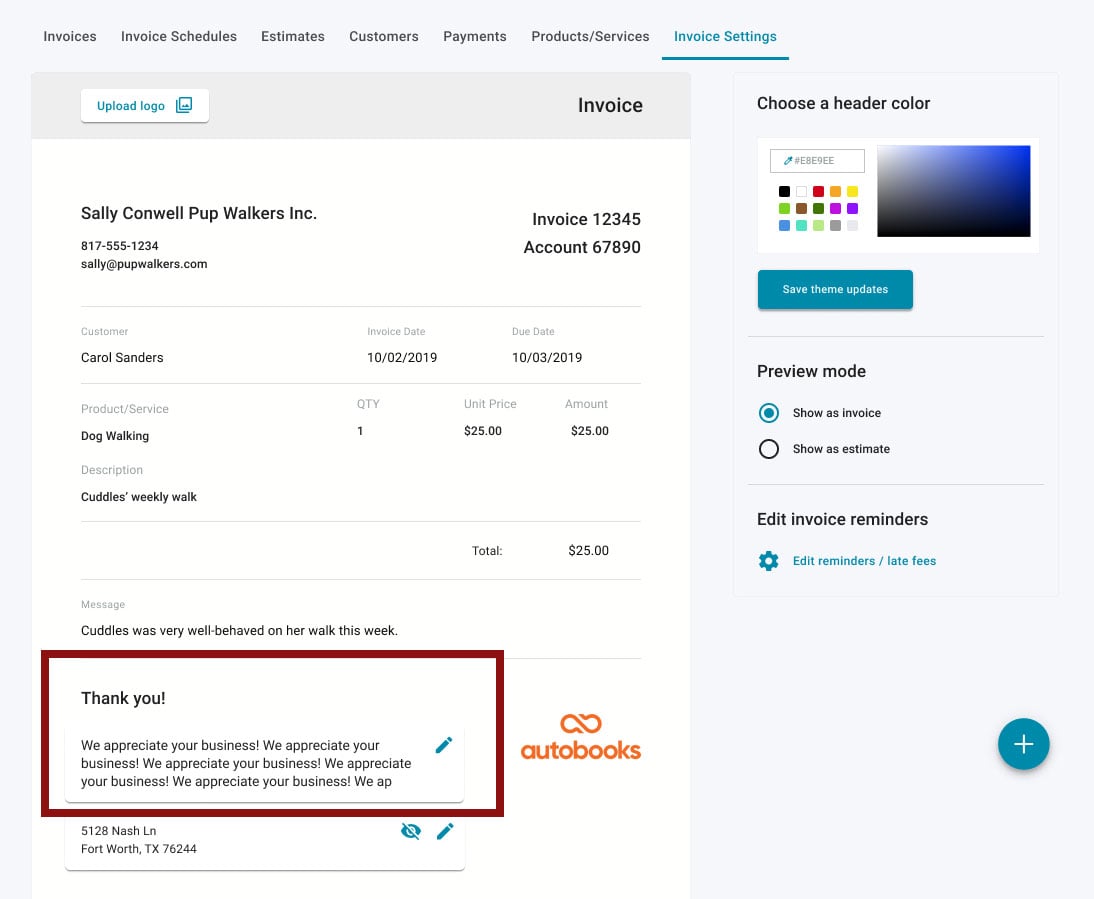This image is a landscape-oriented screenshot depicting an app's settings interface focused on invoice management. The main frame of the app features a dominant blue background with a smaller white box centered within it. 

At the top of the screen, a horizontal navigation menu displays several options in black font: "Invoices," "Invoice Schedules," "Estimates," "Customers," "Payments," "Product Services," and "Invoice Settings." The "Invoice Settings" option is highlighted in blue with a greenish-blue underline indicating it is currently selected.

On the left side, there's a long, rectangular gray box with a nested white box inside. This white box contains green text reading "Upload Logo," and the word "Invoice" appears in black lettering to its right.

Below this, the information for "Sally Conwell Pupwalkers, Inc." is displayed in a white box. This section includes a phone number and email address, followed by details such as an invoice number and an account number.

The layout is sectioned off with gray borders, creating distinct areas for different categories. The first section lists the Customer as "Carol Sanders" and the Product/Service as "Dog Walking." The Description box notes "Cuddles Weekly Walk," and the invoice amount is shown to be $24.

At the bottom of the screen, there is a message stating, "Cuddles was very well-behaved on her walk this week." Adjacent to this, a thank-you note in a red-bordered box reads, "We appreciate your business."

To the far right, an orange icon labeled "Autobooks" is visible, indicating the app or service used for these invoice settings.